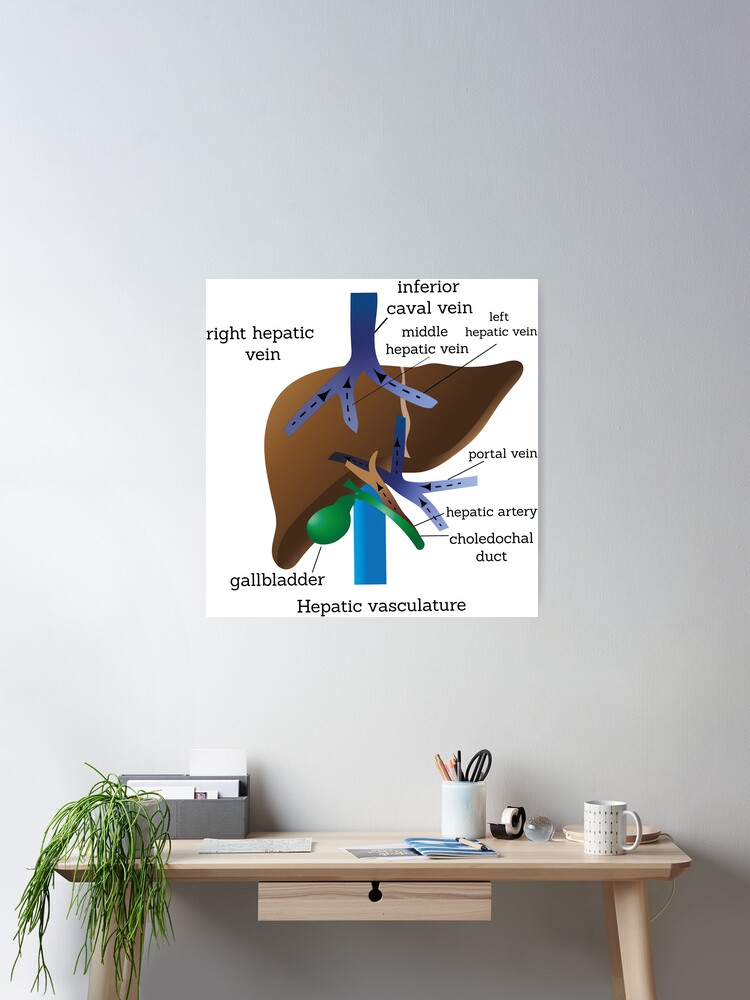The image depicts a small, light wood-colored desk positioned towards the bottom right and center of the frame. On the desk's far left edge sits a single plant. Behind it, against a wall that transitions from bright white to gray as it rises, there is a gray container. This wall appears white on the bottom left, gradually fading to gray towards the upper right due to a light source from the bottom left. The desk features a variety of items: a white container filled with pencils and scissors, a tape dispenser, a coffee mug, and a white table lamp. Scattered papers indicate active use, while an under-desk drawer offers additional storage. Above the desk, a poster labeled "Hepatic Vasculature" displays a detailed diagram of liver anatomy, including the gallbladder, right hepatic vein, interior vena cava, middle hepatic vein, portal vein, and hepatic artery. This setup suggests a medical or research environment, highlighting both functional workspace elements and specialized anatomical reference material.